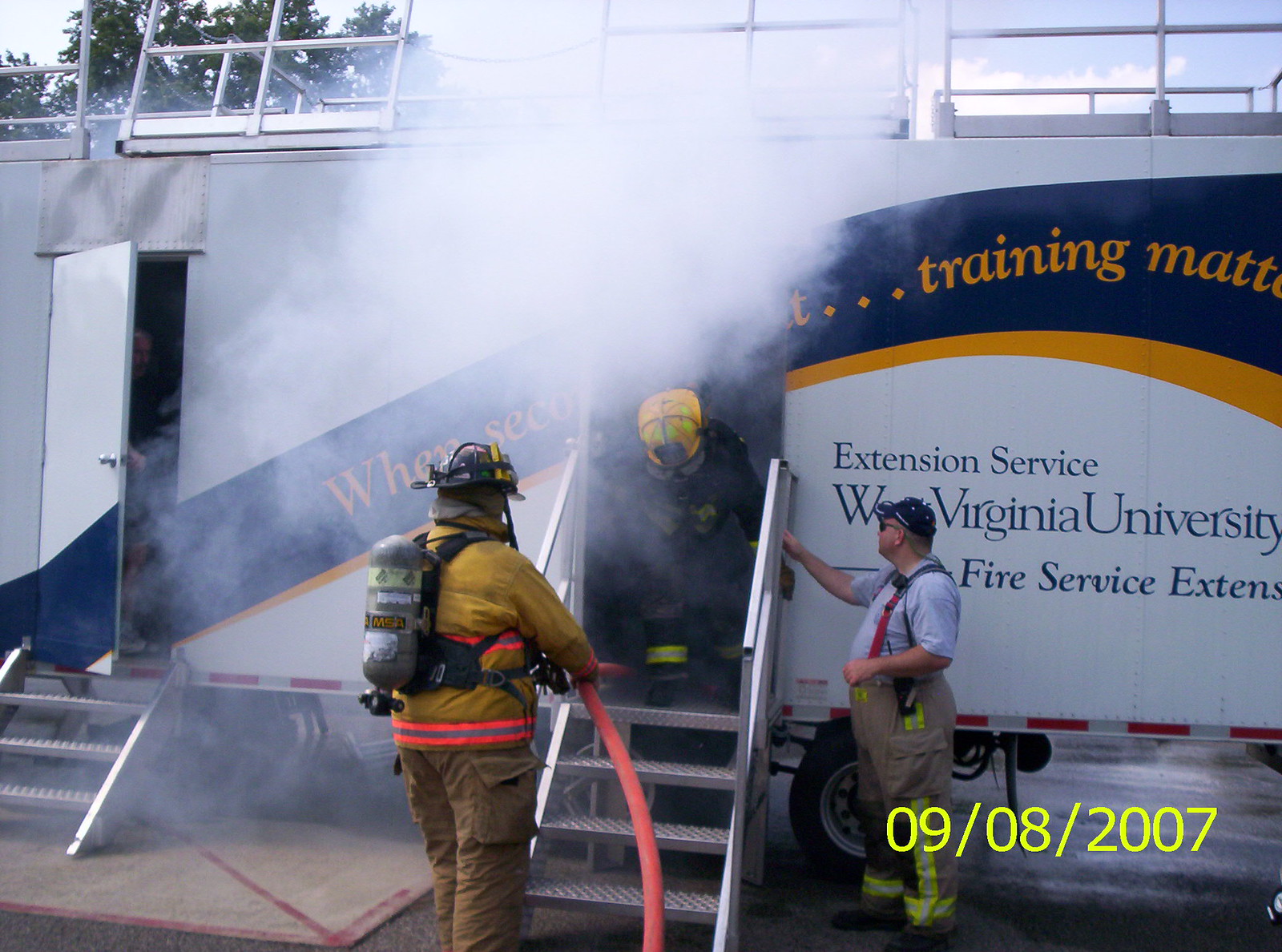The image depicts three men around a mobile training unit, which appears to be a tractor-trailer, likely used for firefighter training. The trailer features metal stairs leading up to it and has smoke billowing out of its right-side doorway, adding a sense of urgency and realism to the training scenario. The trailer is marked with several partially obscured words, including "WHEN...TRAINING," "EXTN SERVICE," "WEST VIRGINIA UNIVERSITY FIRE SERVICE." A date, "09/08/2007," is visible in the bottom right corner.

One man, positioned at the doorway window of the trailer, is hunched over and wears a blue fire helmet. Another man stands to the left in full firefighter gear, including a yellow helmet, a reflective jacket, pants with cargo pockets, and an oxygen tank on his back. He holds a red hose, ready for action. The third man, situated on the right, wears a blue hat, a gray t-shirt, and firefighter pants with reflective strips. The scene is set against a backdrop of a blue sky and trees, emphasizing the training environment’s location.